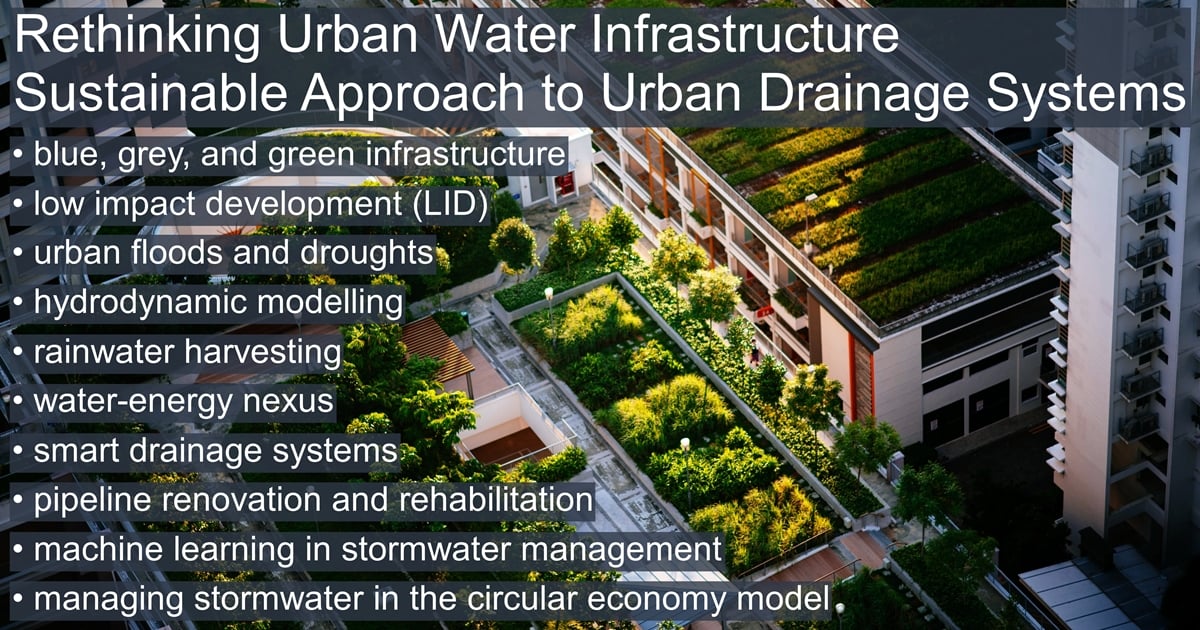The image is a detailed poster focused on sustainable urban water management. It features white text overlaid on a background photograph depicting a cityscape with multiple buildings, including a large institutional-looking building and high-rise apartment buildings with rooftop gardens. The scene also includes a sunlit plaza with organized rectangular plots of greenery and trees, emphasizing the integration of vegetation in urban areas.

The poster is titled "Rethinking Urban Water Infrastructure" and "Sustainable Approach to Urban Drainage Systems." It lists several key points in bullet form:
- Blue, Gray, and Green Infrastructure
- Low Impact Development (LID)
- Urban Floods and Droughts
- Hydrodynamic Modeling
- Rainwater Harvesting
- Water Energy Nexus
- Urban Drainage Systems
- Pipeline Renovation and Rehabilitation
- Machine Learning in Stormwater Management
- Managing Stormwater in the Circular Economy Model

The overall theme of the poster emphasizes innovative and sustainable methods for managing urban water systems, integrating technology, and green infrastructure to enhance city resilience.